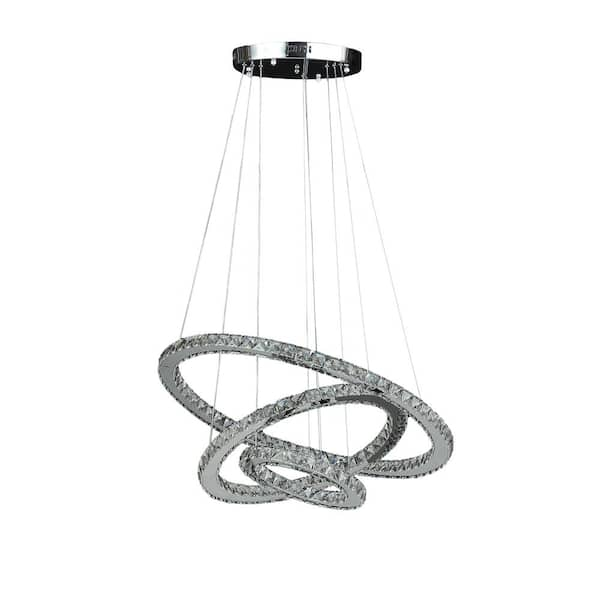This image features an intricately designed modern chandelier set against a pure white background, likely showcased as an online product. The chandelier boasts a sleek chrome finish and comprises three graduated circular tiers of varying sizes, each suspended from a central chrome stem leading up to the ceiling. These tiers are accented with strands of crystals that hang elegantly from each ring, reflecting light and adding a touch of sparkle. The smallest ring is situated in the middle, the second tier is slightly larger and appears tilted at a diagonal angle, while the largest ring encapsulates the other two, also tilted in another direction. Thin, almost invisible wires delicately connect each ring to the chrome stem, giving the chandelier a floating, ethereal quality. The overall design exudes a contemporary and sophisticated aesthetic, intended to offer a sleek and modern look for potential buyers evaluating this item either online or in person. Photographed with professional lighting and a minimalist background, the chandelier's shiny, jeweled surfaces and finely detailed craftsmanship are prominently highlighted.